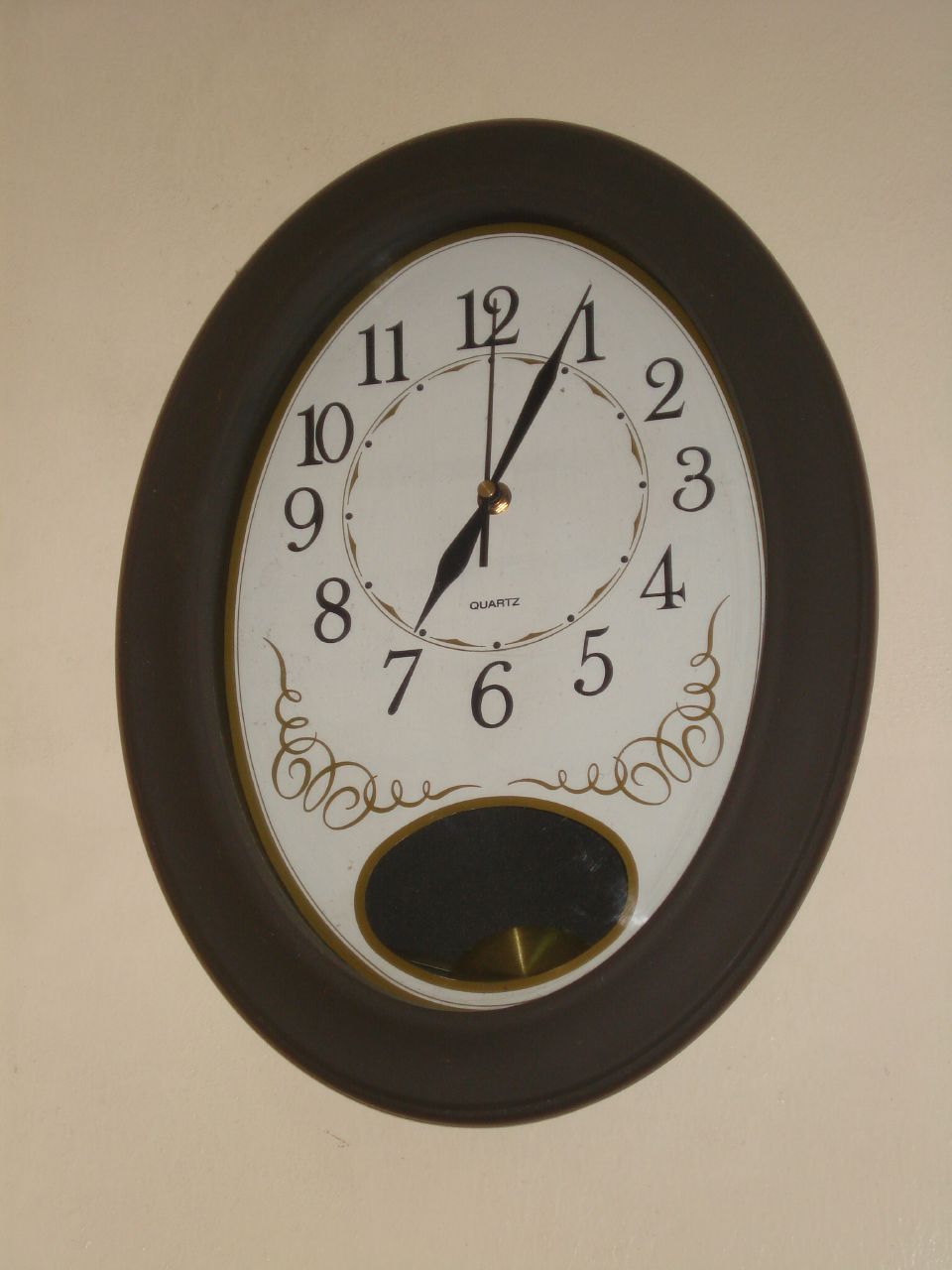The image features a clock with a white background. The main face of the clock is a black circle, while an additional white circle is positioned within it. This white circle has a curved, ornate design, and at the bottom of the face, there is a circular pattern. Encircling these elements is a detailed border with dots connected by a round line pattern. 

The clock face is designed to mimic the appearance of an hour hand pointing at 7 o'clock, a minute hand pointing at 1 o'clock, and a second hand pointing directly at 12 o'clock, all anchored by a central metal pin. Below the clock face, near the 6 o'clock position, is the word "Quartz."

Towards the bottom of the black circle, there appears to be a window showing a pendulum mechanism in motion. This lower portion is styled to look like another black circle, creating a layered visual effect.